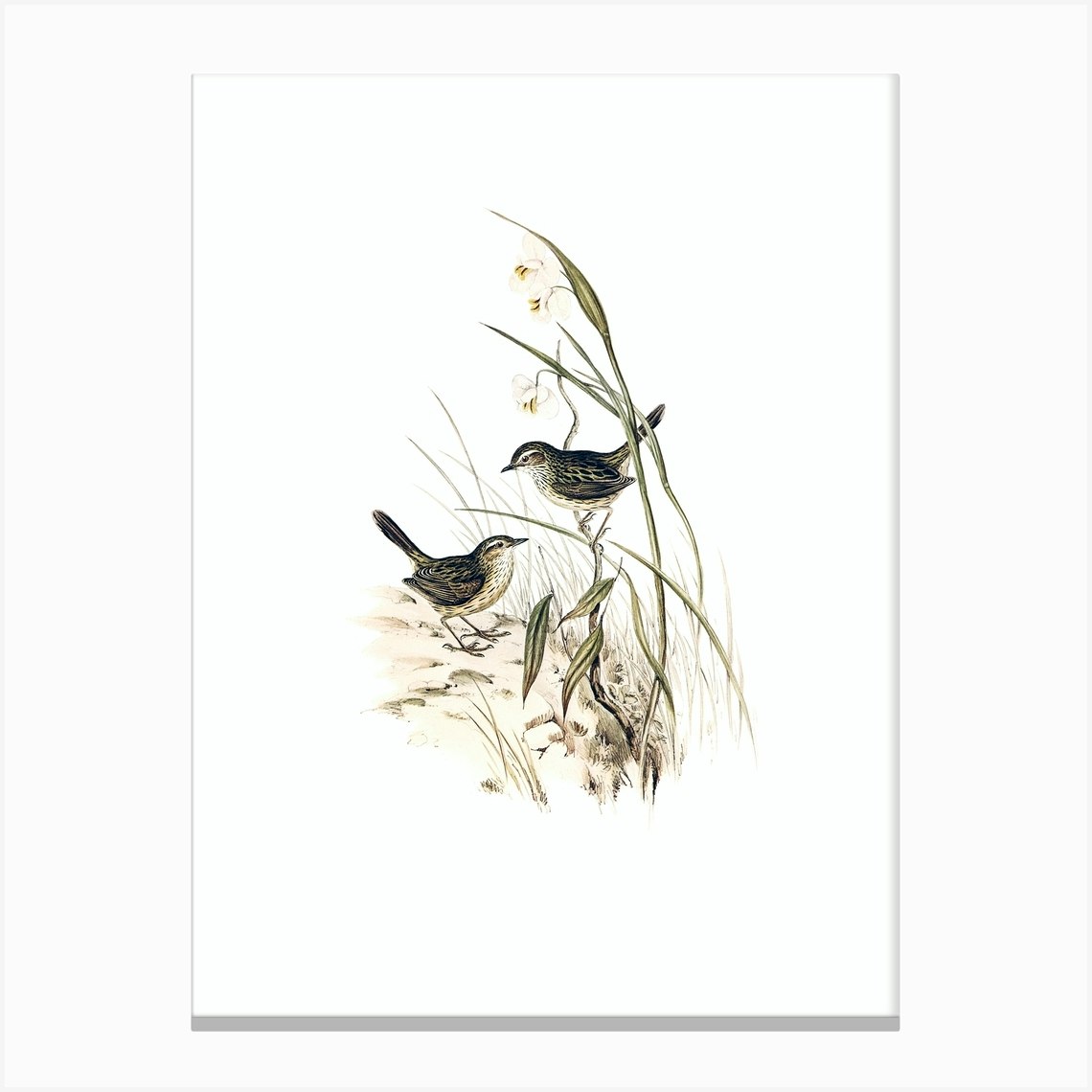The image depicts a minimalist sketch set against a white background, with all elements concentrated in the center, leaving ample white space around. The focal point features two birds, resembling sparrows, interacting with each other. One bird is perched on a tall gray and tan stem that resembles dried grass on the right side, while the other bird stands on the ground, marked by light gray sketch lines to illustrate dirt and leaves. The bird on the branch, which has a brown head and looks slightly downward, appears to be gazing at the second bird on the ground. This bird on the ground, slightly larger and showing its white speckled chest and brown back, looks upwards towards the perched bird. The illustration includes some green stems and small brownish flowers, contributing to the naturalistic setting. Both birds have distinct markings, with white underparts speckled with black, dark brown upper parts, and eyes accentuated by white backgrounds.